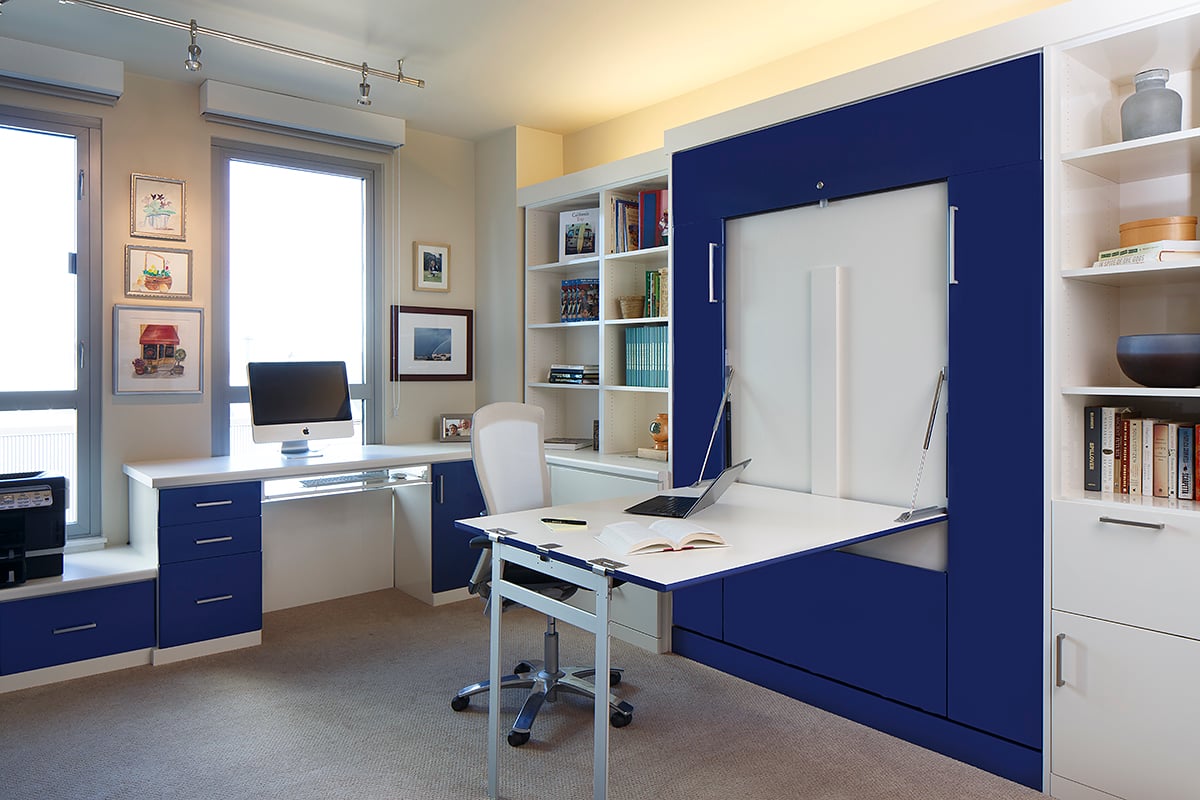This image captures a bright and modern office environment, likely a home office, characterized by a cohesive blue and white color scheme. The centerpiece is a blue desk with a white tabletop, featuring an Apple computer screen positioned near two tall windows that offer an outside view. This office also includes a cleverly designed fold-down desk that extends from the wall, resembling the mechanism of a Murphy bed, and it holds a laptop, an open book, and a pen. Above this innovative desk space, the dark blue wall is flanked by built-in shelves housing books, vases, and other decorative items. The office space is thoughtfully illuminated with a combination of recessed lighting above the bookshelves and modern rail lighting on the ceiling. Framed drawings adorn the walls, adding to the aesthetic appeal. A sleek, white chair with wheels sits in front of the desk, enhancing the overall sense of a tidy, functional, and inviting workspace.